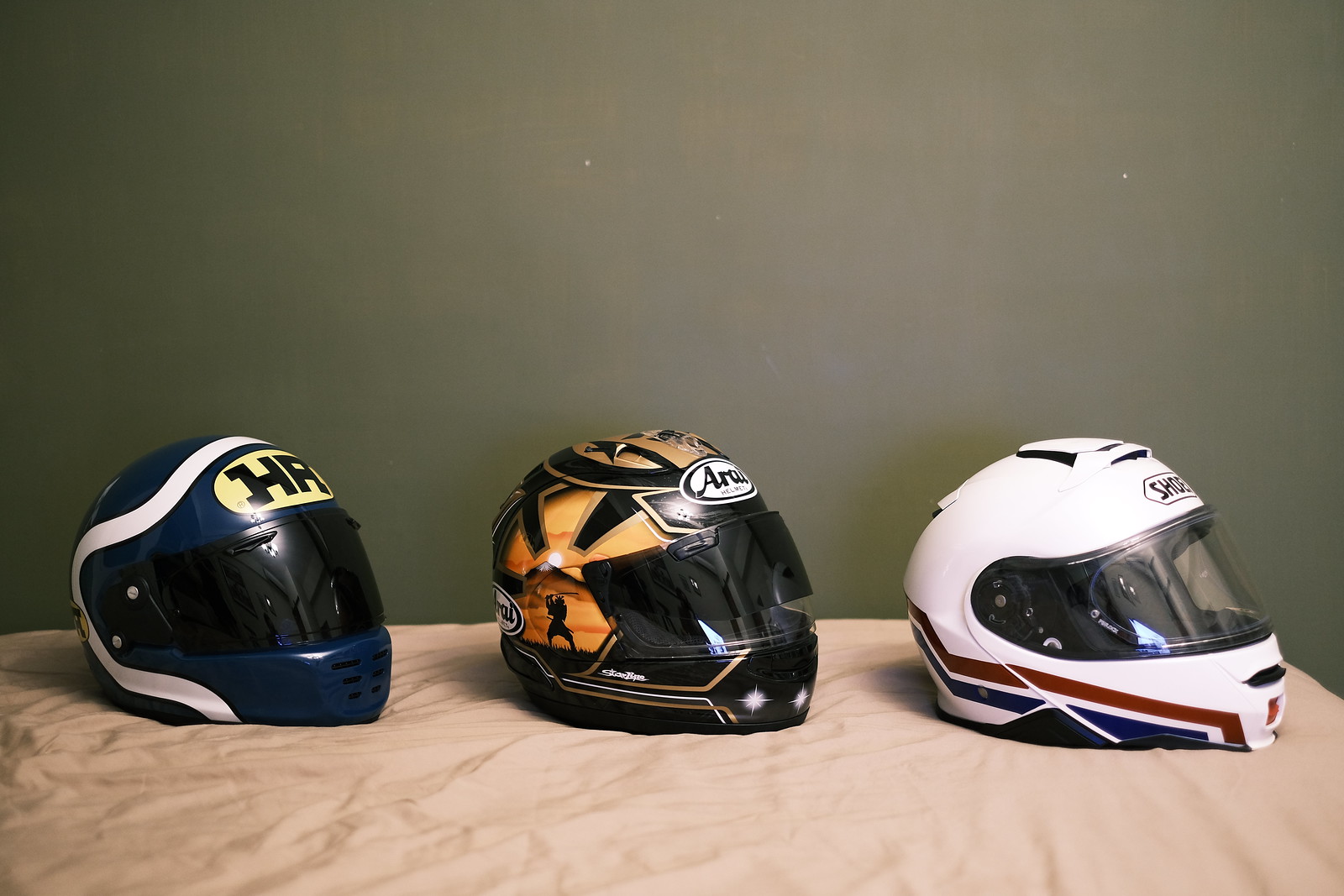This is an image featuring three helmets, presumably designed for motorcycle or racing use, displayed against a dark taupe or dark gray wall and resting on a beige, wrinkled sheet draped over a light brown wooden surface. All helmets have an enclosed front with a wind visor and are angled towards the right-hand side. The helmet on the right is predominantly white with maroon and navy racing stripes on the side and some unreadable text above the visor. The middle helmet is black adorned with orange and gold patches, displaying a silhouette of a human figure against an orange background. The helmet on the left is dark navy blue, featuring a prominent white stripe and a yellow oval with black letters "HR" on its front.